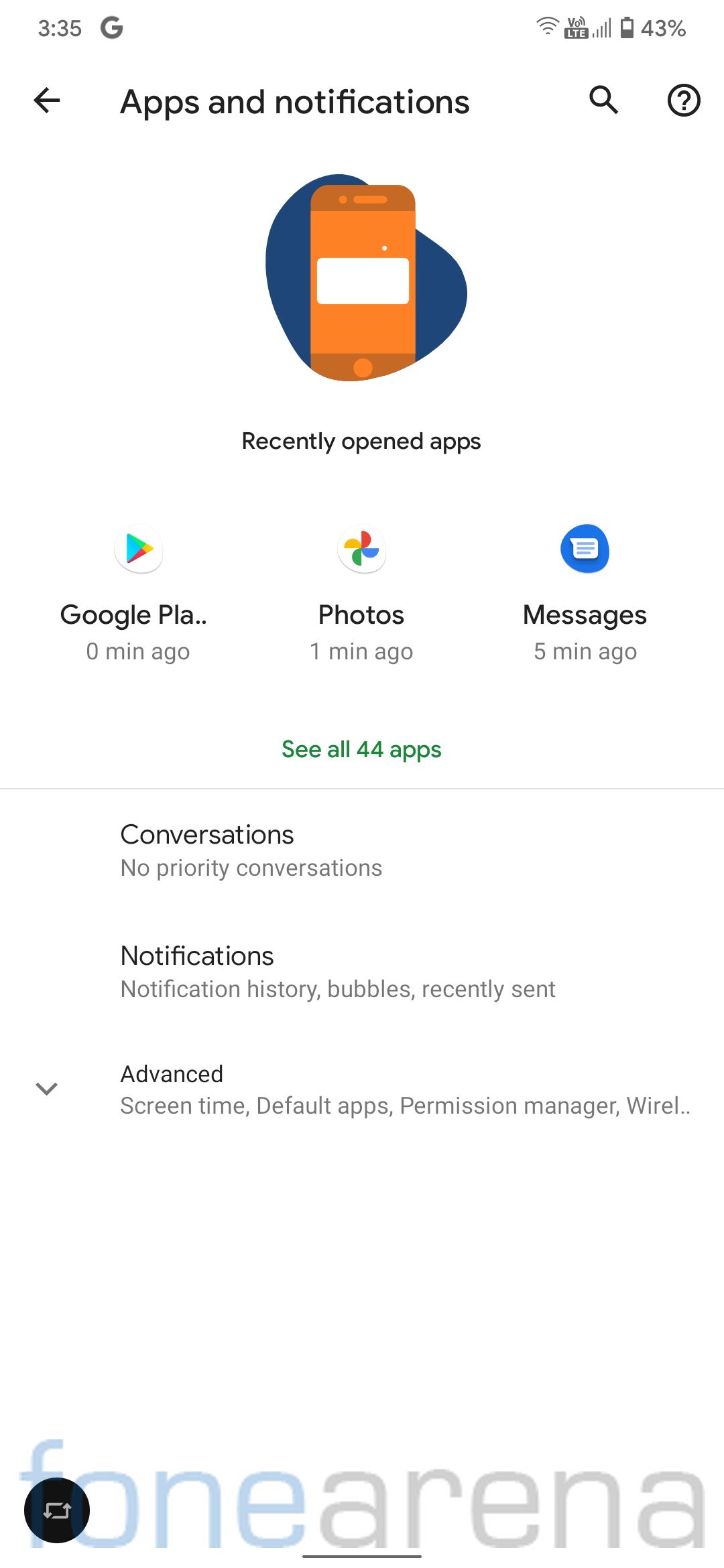This image is a detailed screenshot from a smartphone with a white background. 

- **Top Status Bar:** 
  - On the left: The time is displayed as 3:35, though it does not specify a.m. or p.m.
  - Center-left: The letter 'G' in the distinct Google font style is visible.
  - On the right: The battery level shows 43% with icons for wireless connection and Wi-Fi.

- **Header:**
  - At the top of the page, in black font, the text reads "Apps and notifications."
  - To the left of this text is a back arrow pointing to the left.
  - On the right side are a search icon and a help icon (a black question mark encased within a black circle).

- **Graphic:**
  - Beneath the header, there is a simplistic graphic resembling an orange box with a rectangular white window and a background element that is blue and somewhat oval-shaped. This graphic might represent a smartphone, but it requires a closer look to discern that clearly.

- **Content Section – Recently Opened Apps:**
  - The section is labeled "Recently opened apps."
  - Displays three entries:
    - Google Play Store (identified by the pyramid-shaped logo in Google colors: blue, green, red, and yellow).
    - Google Photos (identified by the Google Photos logo).
    - Messages.

- **Footer Links:**
  - In green font, a link reads "See all 44 apps."
  - Another section on the left labeled "Conversations" states there are "No priority conversations" and includes a range of topics: notification history, bubbles, and recently sent notifications.

- **Subcategories:**
  - The "Advanced" section includes:
    - Screen time
    - Default apps
    - Permission manager
    - Partially visible text which likely says "Wireless" (only "Wire" and an 'L' are visible).

- **Watermark:**
  - At the very bottom, in very light font and lowercase, is a watermark probably from the stock photo agency, reading "fonearena."

This descriptive caption gives a comprehensive overview of the elements present in the smartphone screenshot.